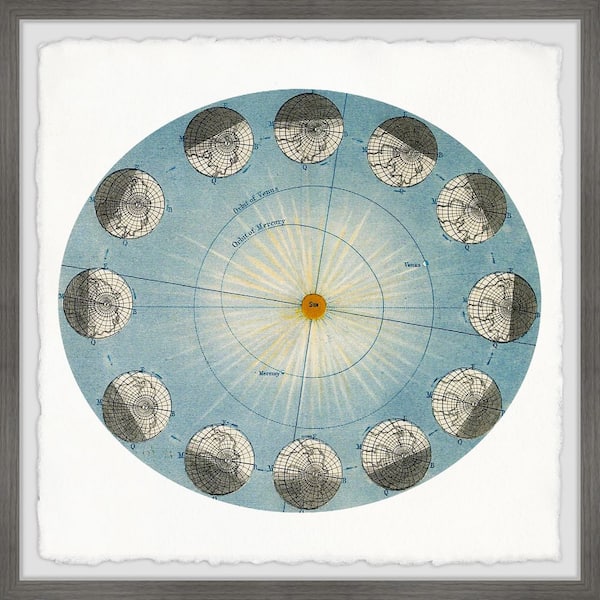The image is an intricate, vintage map illustrating early astronomy with a heliocentric model. At the center is a small, fiery ball labeled "Sun," with rays emanating outward. Surrounding the sun are distinct orbits, labeled for Mercury and Venus, drawn as ovals and circles. The map depicts the Earth eleven times, showing different globe configurations with directional arrows indicating movement and light illumination illustrating the sun's effect on various hemispheres throughout the year. 

The map, printed on a white canvas, appears both historical and detailed, suggesting it might be from the 1700s or 1800s. The background features a white square framed in light gray, encased in a dark charcoal frame, giving it a product-like, display quality. Some elements suggest a blend of antique and modern design, possibly computer-generated, including blue and golden-yellow circles that hint at the equator and lines of direction, and a focal point marked by a golden sun at the center.